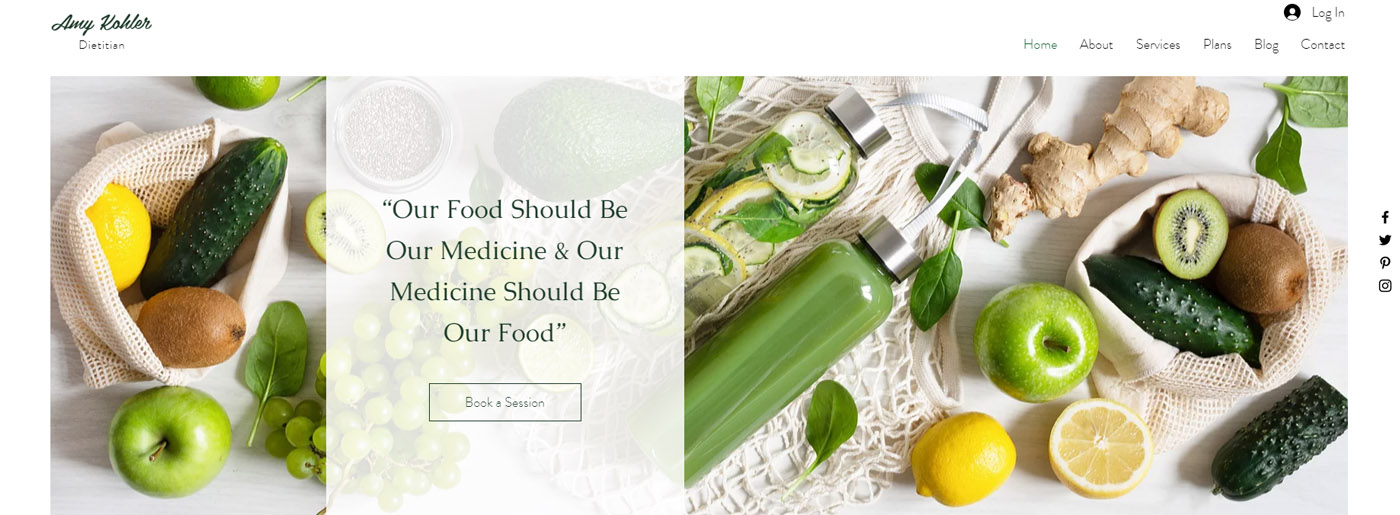The image showcases a vibrant assortment of fresh produce and health-focused elements set against a pristine white tablecloth. Dominating the scene are a variety of fruits and vegetables, including a sliced lemon in the bottom left, a cucumber featuring green spots, a kiwi, an apple at the center, and some ginger root. The top-right and center portions of the image are adorned with lush green leaves, adding to the fresh and healthy aesthetic. 

On the left, there's a bottle filled with a mysterious blue liquid, topped with a silver cap and equipped with a straw. Overlaying the produce, a prominent text reads, "Our food should be our medicine and our medicine should be our food," emphasizing a holistic approach to wellness. Above this message, there are menu options for what appears to be a website, listing "Home," "About," "Services," "Plans," "Blog," and "Contact," along with a call-to-action button "Book a Session."

In the background, a net lightly cradles some of the fruits, adding a rustic touch to the composition. The overall image exudes a harmonious blend of nature's bounty and a contemporary call to health and wellness.